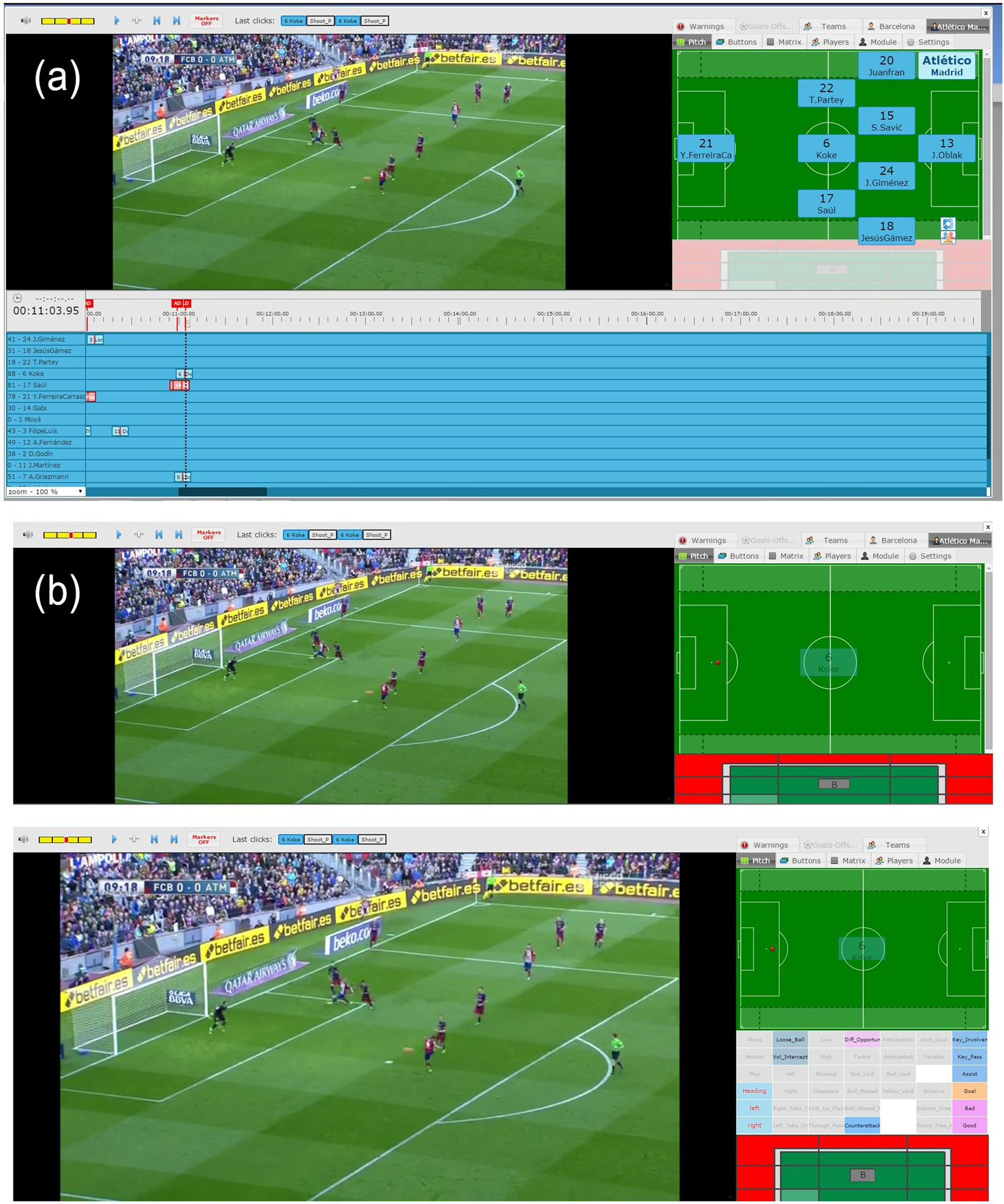The image comprises three distinct screenshots taken from a computer program, aligned horizontally as rows. The top screenshot is labeled with a lowercase "a" in parentheses in the top left corner, the middle screenshot bears a lowercase "b" in parentheses, while the bottom screenshot is unmarked. The content of the screenshots suggests it is a software used for analyzing a soccer match.

In each screenshot, the left half displays a live video feed of the soccer game. The right half of the screen provides a variety of analytical tools. In the uppermost screenshot (a), we see positions of the players marked on a sky view diagram of the soccer field. Additionally, there's a grid that might be outlining game events or moments in time. The user interface is visible at the top, showing a gray bar with a few unidentifiable buttons and a close (X) button in the top right corner.

The middle screenshot (b) continues this format with a similar view of the field. However, this time the pitch is devoid of any player markings, showing only the layout of the field itself.

The bottom screenshot mimics the layout of the first two but without the alphabetical watermark. It shows a clear field from the same angle and lists various items below the field, some of which are activated while others are grayed out, perhaps indicating different states or events during the game.

Overall, the image depicts the interface of a soccer analysis software, possibly used for coaching or game review, including live video, player positioning, and game event tracking functionalities.